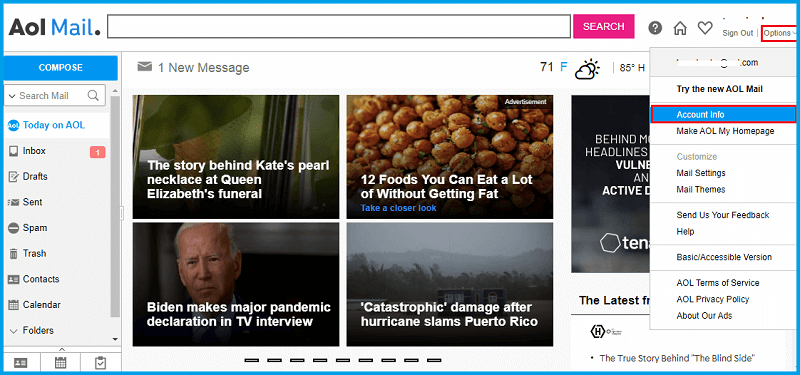Screenshot of AOL Mail Interface

The screenshot captures the AOL Mail interface in detail. The top left displays "AOL" in black and "Mail" in blue, followed by a black dot. To the right, there's a search box and a pink button labeled "Search" in white text. Further right, icons for a question mark, house, heart, and buttons for "Sign Out" and "Options" are visible. The "Options" button is distinguished by a red square border.

Beneath "AOL Mail," a blue button labeled "Compose" with white text appears, followed by "Search Mail" accompanied by a magnifying glass icon. Below this section in blue, "Today on AOL" is displayed, featuring various symbols next to the following categories in black: Inbox (with a red "1" indicating one new message), Drafts, Sent, Spam, Trash, Contacts, Calendar, and Folders.

A notification at the top states there's one new message with an envelope icon below the search box. Further right, the weather is shown: 71°F, partly cloudy, and attributed to Friday night. An displayed icon features a sun partially hidden by a cloud, and 85°F is highlighted as the high.

A section encourages users to "Try the new AOL Mail" in black text with "account info" in blue and boxed in red below it. Additional options include "Make AOL my home page" in black, "Customize" in gray, followed by "Mail settings," "Mail themes," "Send us feedback," "Help," "Basic accessible version," "AOL terms of service," "AOL privacy policy," and "About our ads."

Centered are four thumbnail images with accompanying headlines:
1. Top left: "The story behind Kate's pearl necklace at Queen Elizabeth's funeral."
2. Top right: "The 12 foods you can eat a lot without getting fat," featuring garbanzo beans in an air fryer.
3. Bottom left: A picture of Biden with the headline "Biden makes major pandemic declaration in TV interview."
4. Bottom right: "Catastrophic damage after hurricane slams Puerto Rico" over an outdoor scene of trees and sky.

Below is a segment starting with "The true story behind The Blind Side," most of which is obscured by a clicked-opened box.